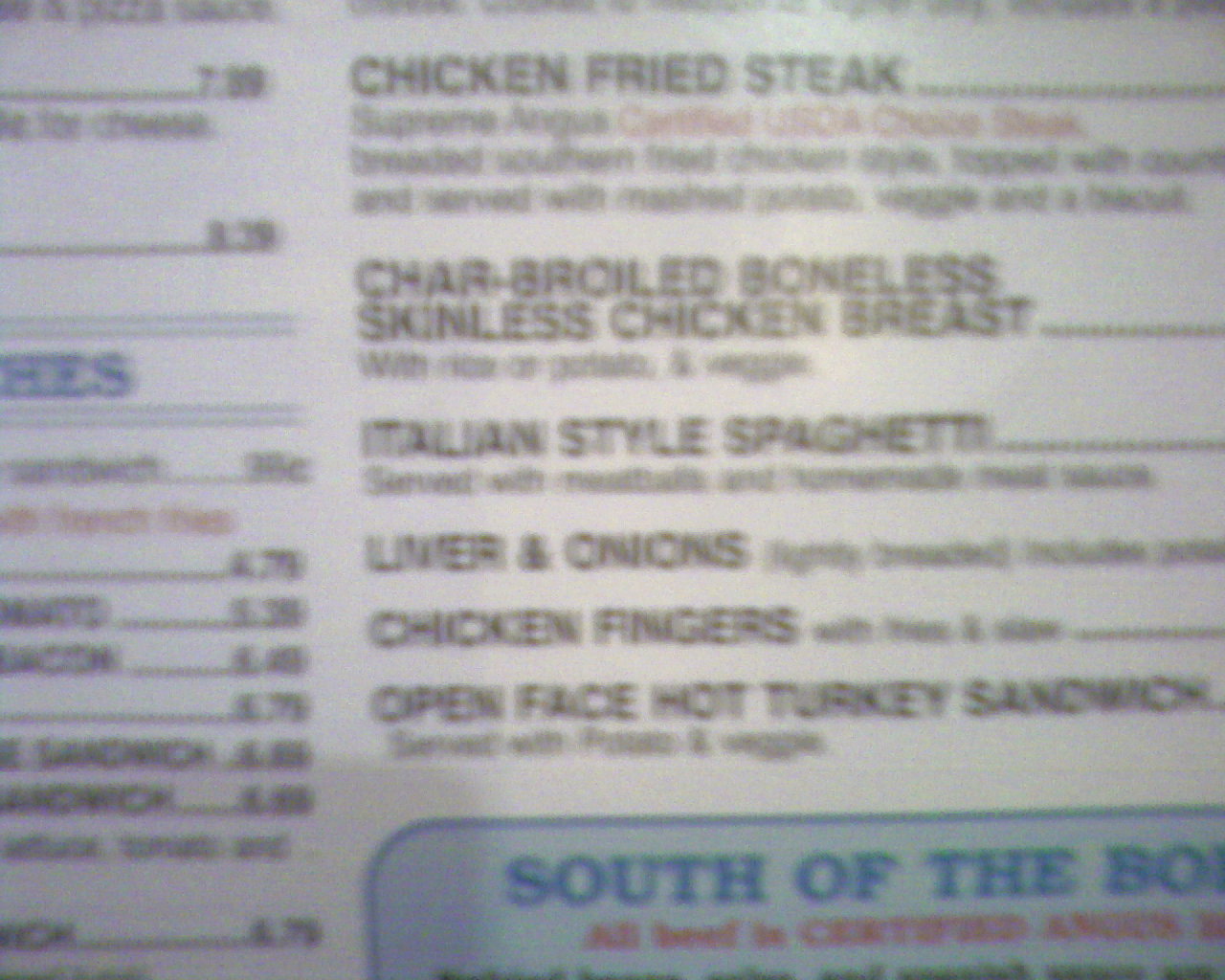This image showcases a partial view of a restaurant menu. The menu is primarily white with black text, accented by blue highlights for certain sections and red for specific words or phrases. The layout features two columns, with the left column partially cut off from view and the right column occupying approximately two-thirds of the visible space.

At the top of the right column, in a bold, larger font, is the item "Chicken Fried Steak." Below this, in smaller black text, is a description that includes the phrase "Certified Something," highlighted in red.

Following the same format, the next menu item listed is "Charbroiled Boneless Skinless Chicken Breast," with a detailed description in smaller black font underneath.

Continuing down the menu, the subsequent items listed in large font are:
- "Italian Style Spaghetti"
- "Liver and Onions"
- "Chicken Fingers"
- "Open Face Hot Turkey Sandwich"

Below these items, within a blue rectangle featuring rounded corners and a lighter blue background, the phrase "SOUTH OF THE B-O" is prominently displayed in all capital letters. The text in this section is in blue font, while additional smaller writing in red appears below it, partially cut off in the image.